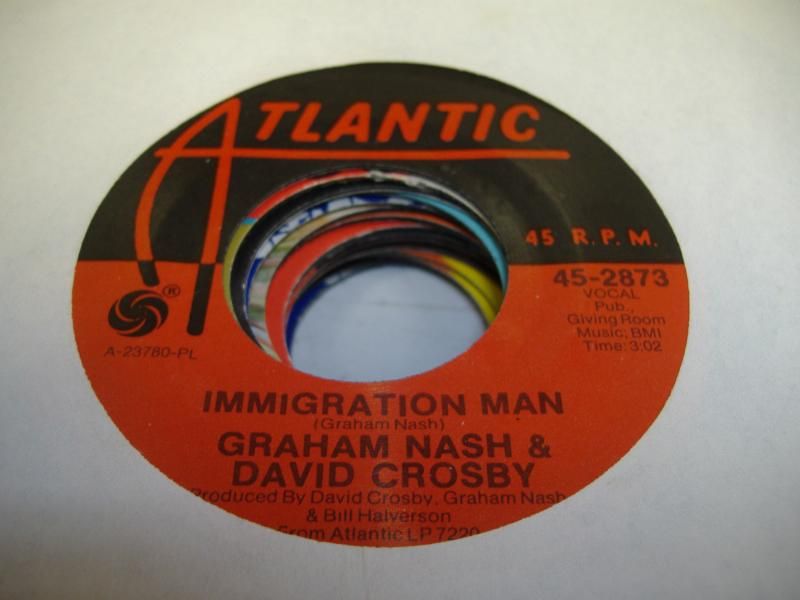The image shows a stack of approximately 12 to 15 vinyl 45 RPM records against a slightly dirty light gray background with yellowish tones. The top record, which is clearly visible, features a distinctive label from Atlantic Records. The label is split into two halves: the upper half is black with "Atlantic" and "45 RPM" written in bold red letters, while the lower half is red with black text. This red section includes details such as the song title "Immigration Man" and the artists Graham Nash and David Crosby. Further information on this section includes production credits to David Crosby, Graham Nash, and Bill Halverson, as well as some cataloging details: "45-2873," "vocal pub and music BMI," and the track's duration of 3:02. Through the central hole of this top record, additional records can be seen stacked beneath, though their details are not readable.